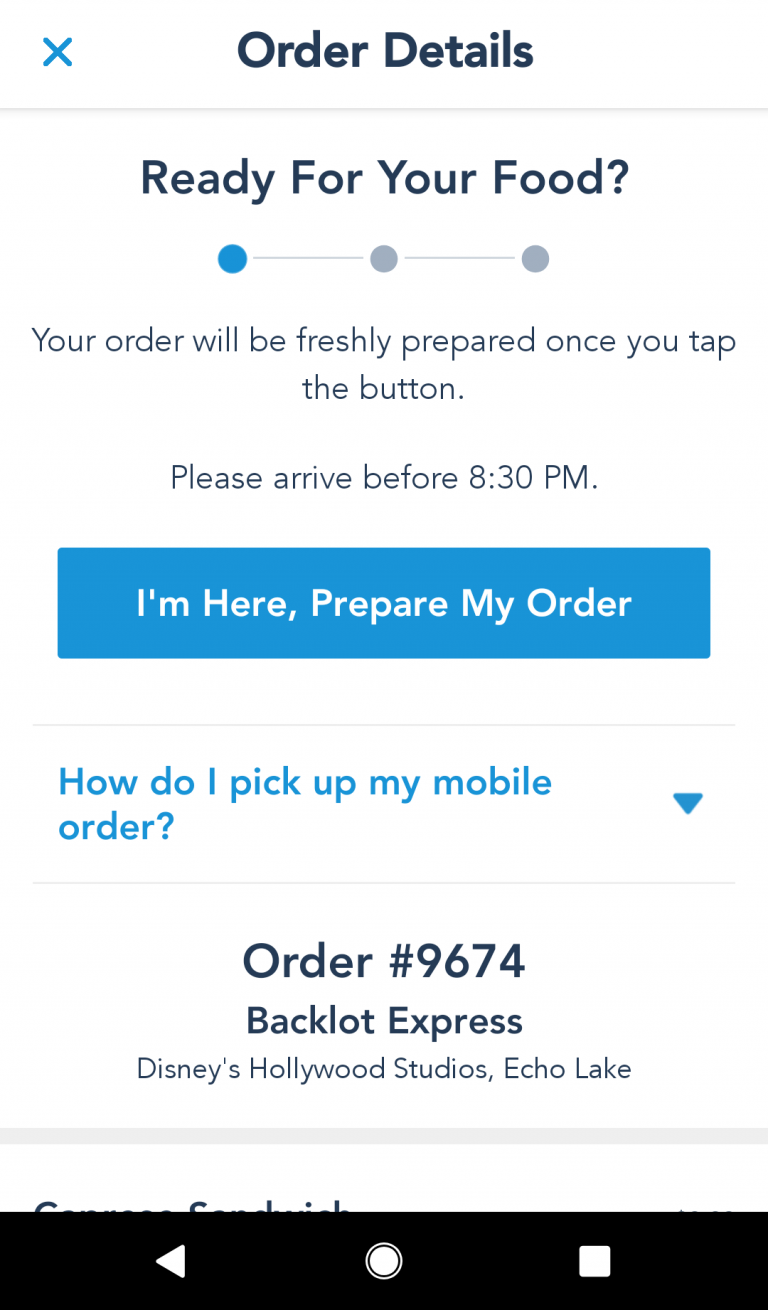The image contains several elements arranged to convey information about a mobile order at a Disney location:

**Top Left:**
- **Text Box 1:** Contains order details.
- **Text Box 2:** Displays the message "Ready for your food."

**Visual Elements:**
- **Blue Circle:** Followed by two grey circles, indicating progress or status.
- **Text Box 3:** Instructs "Your order will be fresh if you're willing to tap the button."
- **Text Box 4:** Advises "Please arrive before 8.30pm."

**Blue Border Section:**
- Contains the prompt "I'm here, prepare my order."

**Dropdown Section:**
- **Question Text:** "How do I pick up my mobile order?"
- Dropdown menu for additional instructions.

**Order Details:**
- **Black Text:** "Order number 9674," location "Backlot Express, Disney's Hollywood Studios, Echo Lake."

**Additional Visual Elements:**
- **White Rectangle:** Contains important information or acts as a divider.
- **Black Bar:** Features a left white triangle, a white circle, and a white square.

**Background:**
- Predominantly white, emphasizing clarity and readability of the text elements.

**Summary of Order:**
- The image is related to mobile order number 9674 at the "Backlot Express" in Disney's Hollywood Studios, Echo Lake area.

This detailed caption aims to provide a clear and organized description of the various elements in the image, catering to a better understanding of its structure and content.